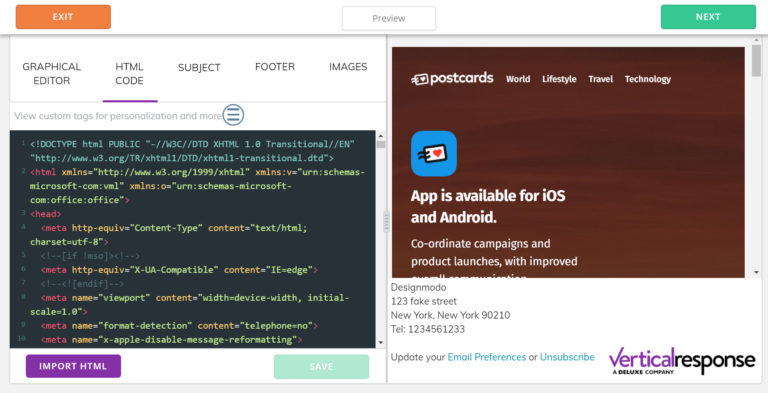The image is of an online code testing platform that allows users to execute and preview their code in real time. The interface is divided into two main sections: the code editor on the left and the live display on the right.

On the left side, the code editor displays a web page's source code, written in a combination of HTML, CSS, and potentially JavaScript. The code includes various elements such as the `<!DOCTYPE html>` declaration, HTML tags, CSS rules, and JavaScript variables and comments, creating a thorough and technical layout typical of web development.

On the right side, the live display shows the result of the executed code, rendering a web page titled "Postcards." The webpage promotes an application available for both iOS and Android, highlighting features like coordinating campaigns and product launches. The background color of the page is brown, and there is placeholder text, likely Lorem Ipsum, filling out the content. An address located in New York is also visible at the bottom of the page. The image succinctly captures the essence of a web development testing environment, demonstrating both the coding process and the resulting web page visually.